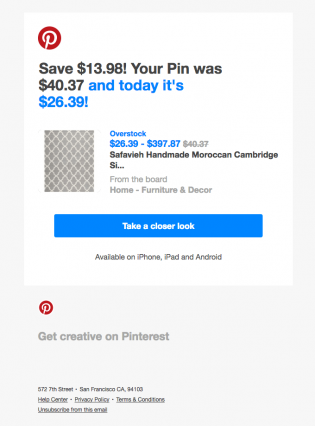This image is a screenshot of a Pinterest banner with a white background. On the top left corner, the iconic Pinterest logo is prominently displayed as a red circle containing a white 'P'. Directly below the logo, black text states, "Save $13.98, your pin was $40.37," followed by blue text reading, "and today it's $26.39." Beneath this, there is an image of a Moroccan Cambridge-style mat. The mat, available from Overstock, is priced between $26.39 and $397.87, and is described as a Savavi, handmade Moroccan Cambridge style decor piece under the home furniture category.

Further down, a blue button with the text "Take a clear look" invites users to explore further. Additionally, small print below the button reads, "Available on iPhone, iPod, and Android." At the very bottom of the banner, additional information includes an address, "San Francisco, California," and several underlined links: "Help Center," "Privacy Center," "Privacy Policy," "Terms and Conditions," and "Unsubscribe from this mail." This detailed layout aims to provide a clear and comprehensive promotional message for potential buyers.